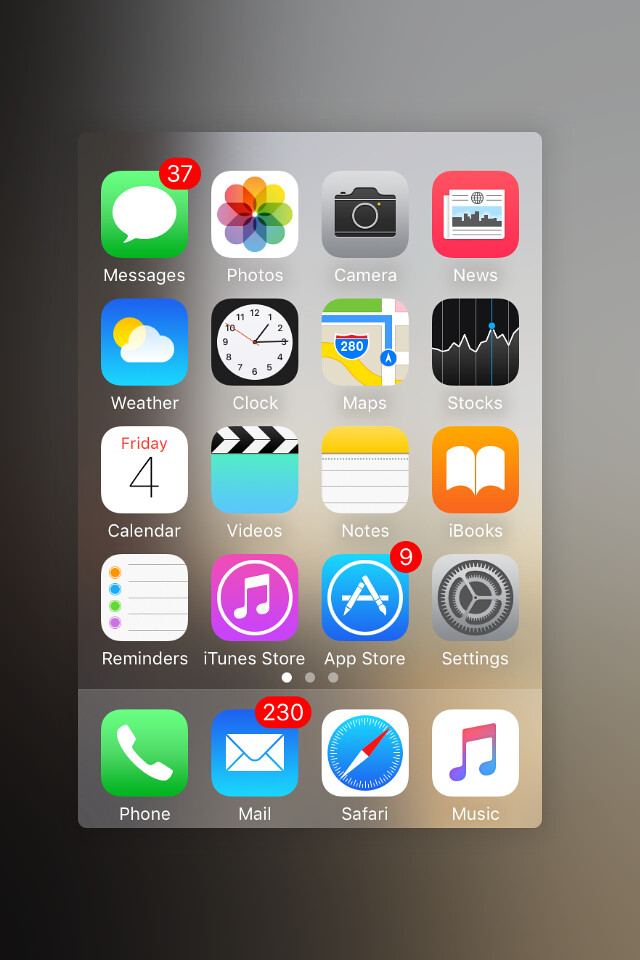**Detailed Caption:**

This image displays an older Android cell phone screen, possibly from a Google device, showcasing a grid of 20 app icons. The screen is neatly organized into five rows, each containing four distinct icons.

- **Top Row, from left to right:**
  1. A green and white Messages icon indicating 37 new notifications within a red bubble.
  2. A Photos icon depicted as a white square with a rainbow-colored flower in the center.
  3. A Camera icon, grey with a black camera symbol in the middle.
  4. A News icon featuring a red background with a white newspaper graphic.

- **Second Row, from left to right:**
  1. A Weather icon with a blue background displaying a bright yellow sun paired with a white cloud.
  2. A Clock icon, black with a white clock face and black numerals.
  3. A Maps icon showing a tan background with a map pathway bearing the I-280 label.
  4. A Stocks icon, black with a blue and white graph.

- **Third Row, from left to right:**
  1. A Calendar icon with a white background revealing the date “Friday the 4th.”
  2. A Videos icon, blue with a black and white clapper board.
  3. A Notes icon, yellow at the top followed by white resembling notebook paper with black lines.
  4. An iBooks icon, orange with a white book emblem.

- **Fourth Row, from left to right:**
  1. A Reminders icon characterized by a checklist graphic.
  2. An iTunes Store icon, purple with white quarter notes.
  3. An App Store icon, blue with a circular design encompassing a white 'A' formed by a pencil and paintbrush.
  4. A Settings icon, gray with a gear wheel.

- **Bottom Row, from left to right:**
  1. A Phone icon with a green background and a white telephone receiver.
  2. A Mail icon, blue background featuring a white envelope with a red notification bubble showing 2,300 messages.
  3. A Safari icon with a white background encircling a blue compass.
  4. A Music icon presenting a white background with pink and blue quarter notes.